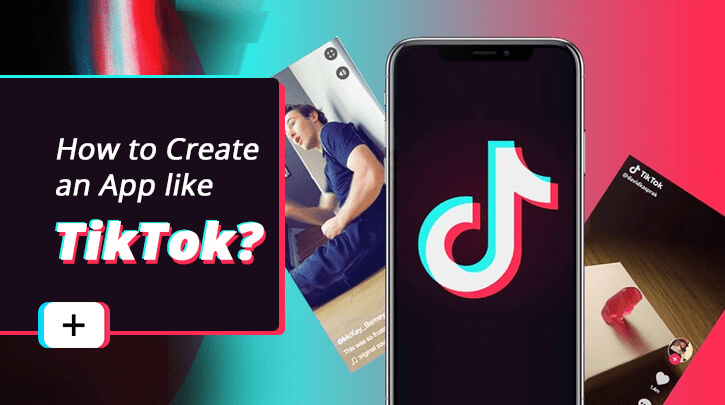This image depicts a detailed advertisement instruction on how to create an app similar to TikTok. The ad prominently features the signature TikTok colors: black, light blue, white, and red. The core of the advertisement contains an image of a phone displaying the TikTok logo. Surrounding the phone, multiple screenshots of TikTok videos are subtly integrated into the background, reinforcing the ad's theme.

On the left side of the ad, there's a black box with bold, white text that reads, "How to create an app like TikTok?" Adjacent to this box, the familiar plus button from the TikTok interface is visible, adding an authentic touch to the advertisement.

Among the screenshots in the background, one shows a man dressed in blue who appears to be surprised, while another depicts a piece of paper on a wooden surface with a gummy bear placed on it, accompanied by a heart icon and indicating that it received 1.4 million likes. The advertisement, rich in TikTok's brand colors and visual elements, clearly serves as a guide or promotional material for developing TikTok-like applications.